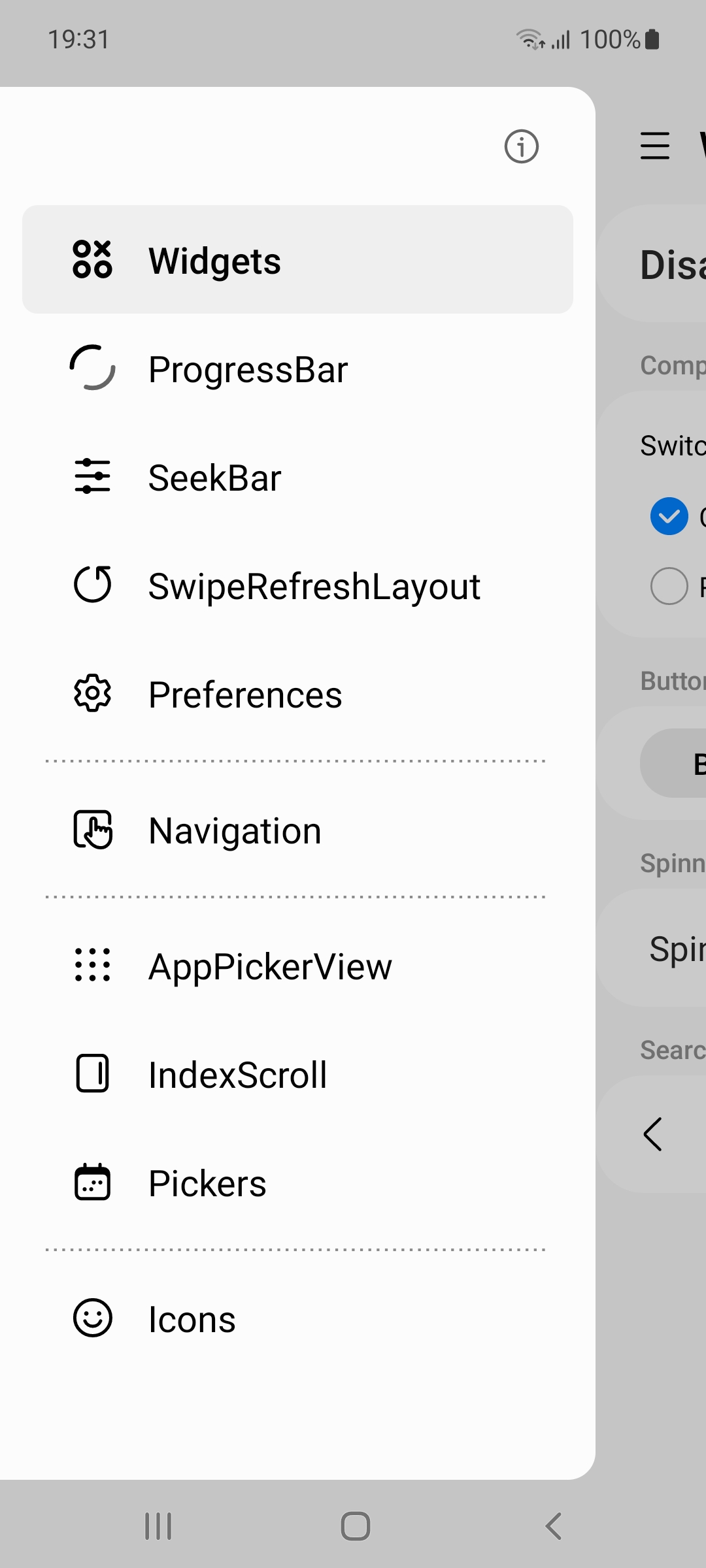Screenshot of a Mobile Interface

The screenshot displays the interface of a cell phone taken at 19:31, as indicated by the time in the upper left-hand corner. The background is a light gray, contributing to a clean and minimalist aesthetic. In the upper right-hand corner, crucial device information such as Wi-Fi reception and battery levels are visible.

Dominating the left side of the screen is a large, open white window that lists various options. To the upper right corner of this window, there is an oval icon outlined in gray, containing a lowercase "i."

The list of options begins with the following entries, each paired with an icon to its left:
1. **Widgets** - This option stands out as it is bolded, indicating it has been selected.
2. **Progress Bar**
3. **Seek Bar**
4. **Swipe Refresh Layout**
5. **Preferences**

A light gray dotted horizontal line separates the subsequent options:
6. **Navigation**
7. **App**
8. **PickerView** (rendered as one word)
9. **Index Scroll** (also rendered as one word)
10. **Pickers**
11. **Icons**

To the right side of the screen, components from the underlying interface are partially visible. The menu bar is discernible along the right edge, with part of the screen below it visible, displaying bold letters "DIS" and fragmented words and buttons. The very bottom of the interface reverts to the light gray background, maintaining the overall design consistency.